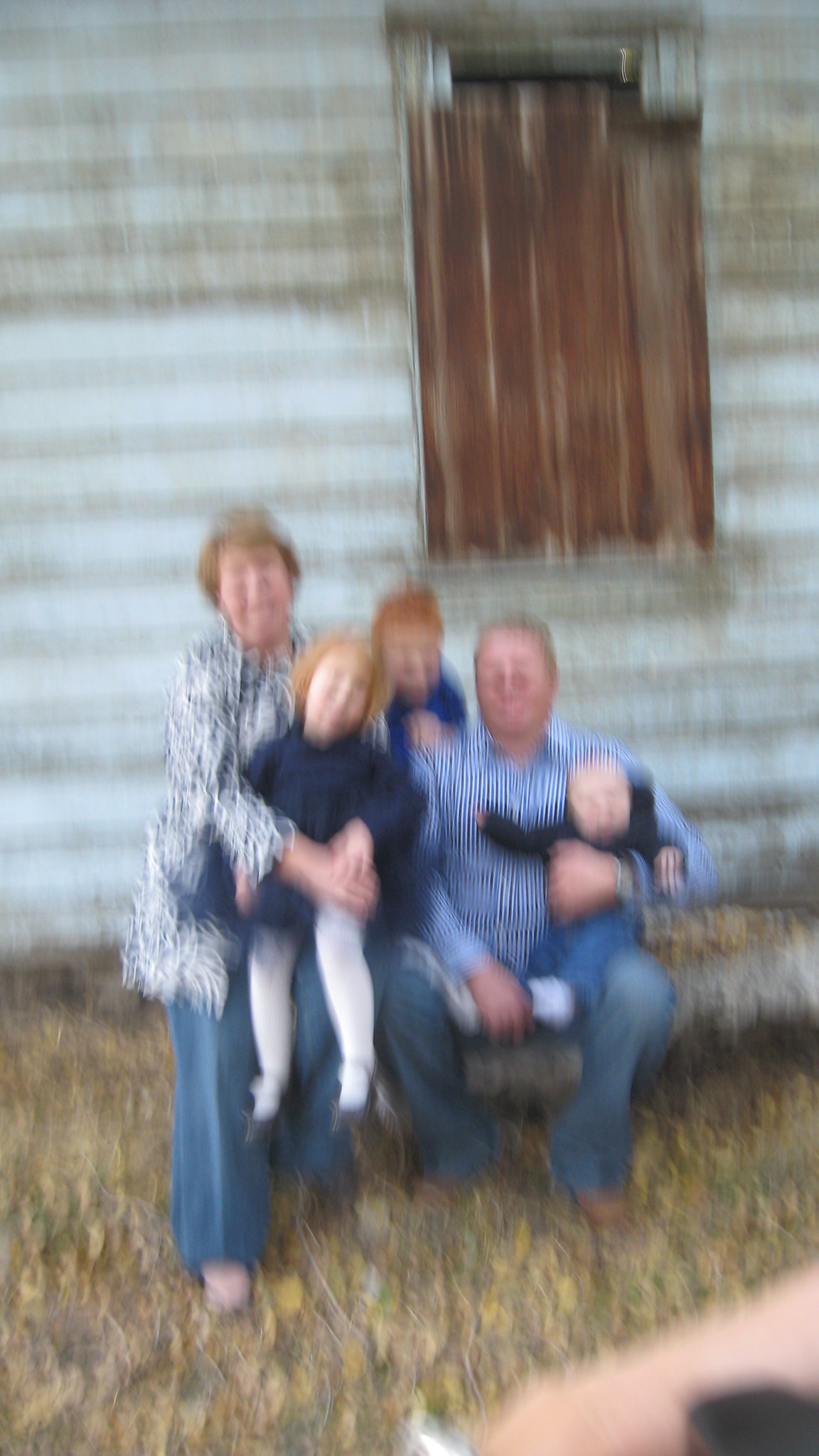In this incredibly blurry photo taken outside, a family of five is seated on a bench in front of a weathered house with horizontal white clapboard siding. The house has a boarded-up window. In the image, on the left, a woman with short brown hair is wearing a long-sleeve blouse with floral designs and blue jeans. Sitting on her lap is a little redheaded girl dressed in a long-sleeved blue shirt and white pants. Just behind the girl stands a young redheaded boy also in a blue shirt. On the right, a man in blue jeans and a white and blue striped long-sleeve shirt cradles a baby with his left arm. The baby is wearing a black long-sleeve shirt and blue jeans. The ground beneath them is covered in leaves. The image is badly out of focus, which makes it difficult to discern finer details.